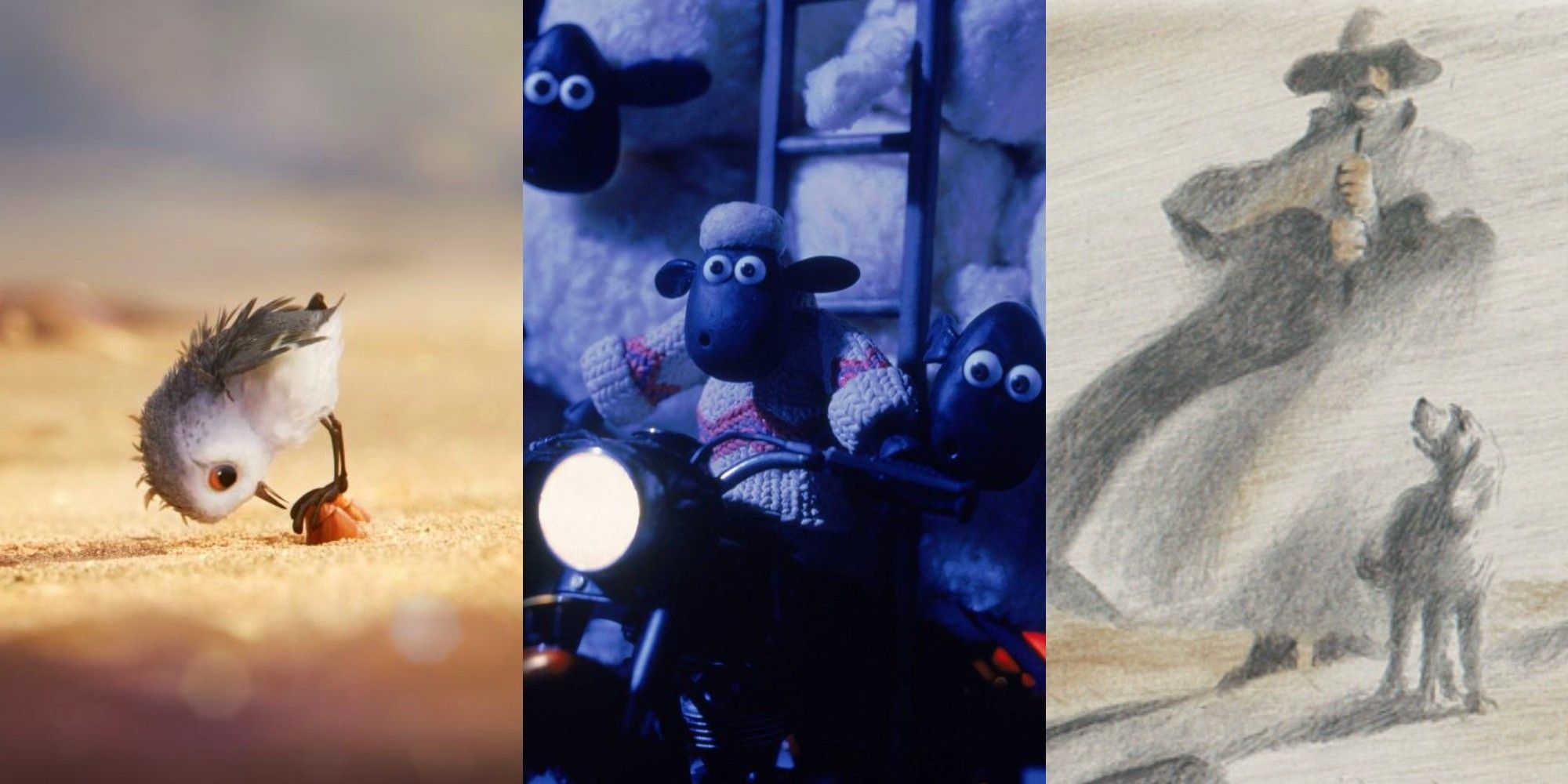The image is a detailed triptych consisting of three separate panels arranged in landscape format. The first panel on the left shows a tiny bird standing precariously on an acorn in a sandy environment. The bird, with gray feathers on its back and white feathers on its belly and face, has its beak pointed towards its feet as if about to crack the acorn. Its feathers appear slightly disheveled, as if wet from a recent storm. In the middle panel, there is a vibrant photo of claymation figures from the movie "Shaun the Sheep." The scene depicts several sheep with black faces and googly eyes, covered in wooly white fur. One sheep, wearing a knit sweater, is driving a motorcycle with another sheep riding on the back, and a comedic plethora of other sheep stacked behind them on a ladder. The motorcycle's headlight is on, illuminating the scene, which seems to be set at night. The third panel on the right features a detailed pencil sketch of a man dressed as a cowboy. He wears a weathered hat with a brim and a long gray overcoat with a cape. He stands holding a staff with both hands, accompanied by a loyal hound gazing up at him. The entire drawing is rendered in shades of gray with subtle tan accents, capturing the serene interaction between the man and his dog.